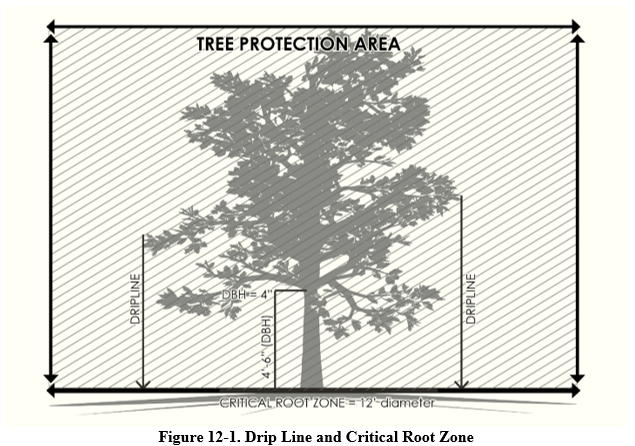The image is a black and white diagram on an off-white background, depicting a large gray silhouette of a tree within a bordered area marked as the "tree protection area." The tree's profile shows several arrows extending from the outermost branches to the ground, labeled as the "drip line," indicating where rainwater drips down from the leaves. Other arrows point to the trunk with a label "4-6 inch DBH," likely referring to the tree's diameter at breast height (DBH). The surrounding border comprises arrows pointing to each corner, highlighting the tree's extent. The area beyond the tree's immediate reach, marked with light gray crosshatched lines, signifies the "critical root zone," specified as having a 12-foot diameter. At the bottom of the image, it reads "Figure 12-1: Drip Line and Critical Root Zone," indicating the diagram’s reference number in a larger publication or textbook.